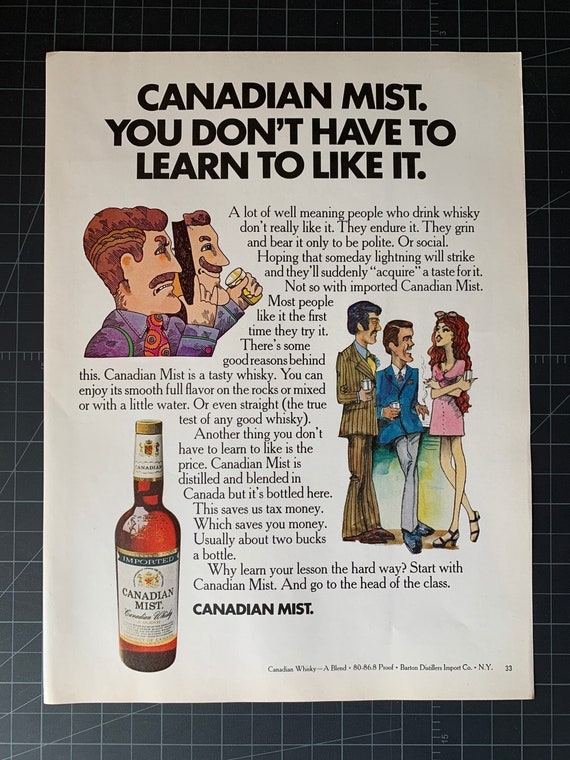This is a full-page magazine advertisement for "Canadian Mist Whiskey," found on page 33, as indicated by the small text in the bottom right corner. The ad features a striking, bold black headline at the top that reads, "Canadian Mist. You don't have to learn to like it." Below the headline, a humorous cartoon illustration depicts a man holding a mask of his own smiling face while his real face underneath shows a frown, suggesting he secretly dislikes the whiskey he's pretending to enjoy.

Adjacent to this illustration, two men in 70s-era suits and ties are seen talking to a young woman in a short pink dress and high heels. The woman is depicted provocatively, emphasizing the social, somewhat risque atmosphere associated with the brand. The men appear to be enjoying the company and drinks, highlighting a social setting where Canadian Mist is featured.

In the lower left corner, there is a detailed illustration of a Canadian Mist whiskey bottle, displaying the amber liquid inside. Running down from the top right of the first cartoon and along the left side of the second cartoon is a lengthy block of text elaborating on the qualities of Canadian Mist and why "you don’t have to learn to like it." The text suggests that many who drink whiskey do so out of social obligation but that Canadian Mist is a whiskey people can genuinely enjoy without pretension.

The ad is laid out on what looks like a black grid or graphing paper background, adding a modern yet classic touch to the overall design. The small print near the page number reads, "Canadian Whiskey, A Blend, 80 86.8 Proof, Bourbon Distillers Import Company, New York."